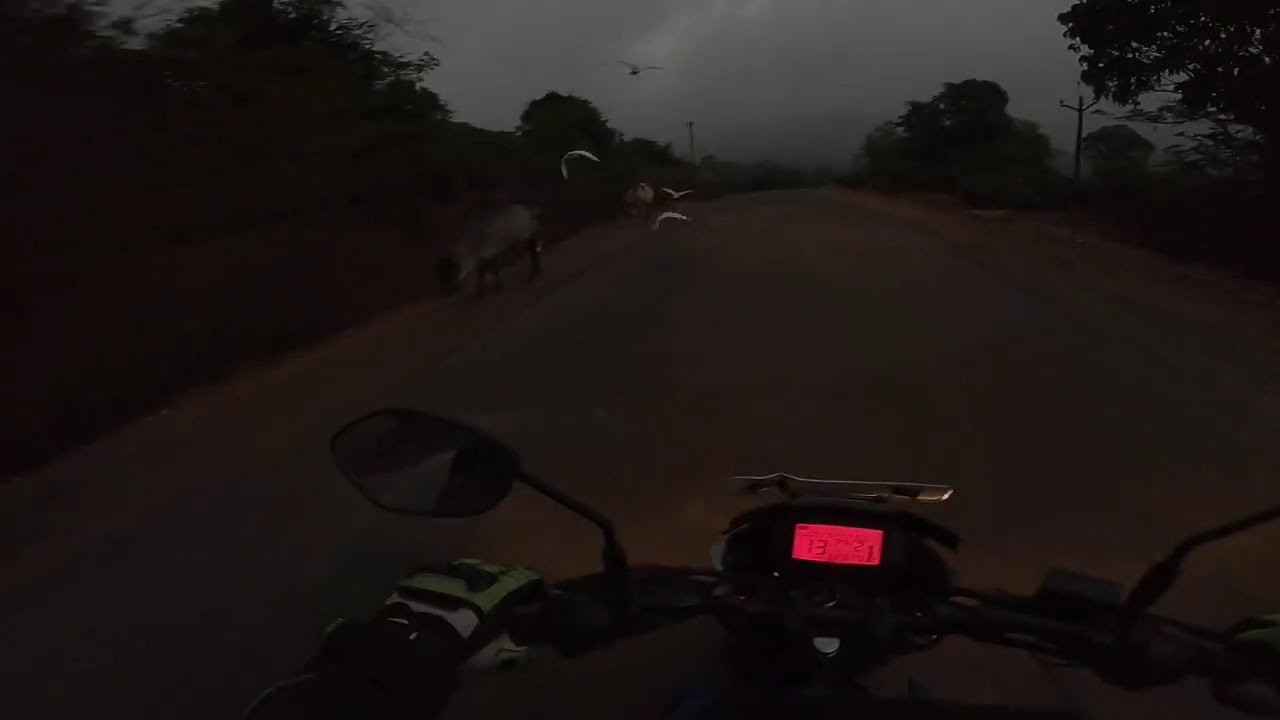In this point-of-view shot, a motorcyclist navigates a mostly sand and dirt-covered countryside road as dusk settles. The dark, cloudy sky casts an ominous hue over the scene, with barely any light except for the red glow emanating from the speedometer on the motorcycle's dash. The rider’s hands, equipped with thick white and yellow gloves, firmly grip the handlebars. The left-hand mirror and a small console displaying red numbers are visible on the motorcycle. Trees flank both sides of the single-lane road. On the right side of the path, a grey-willed beast, possibly a cow or boar, roams while several white birds swoop low past the motorcyclist. The overall atmosphere is dark and misty, contributing to the grainy texture of the image.